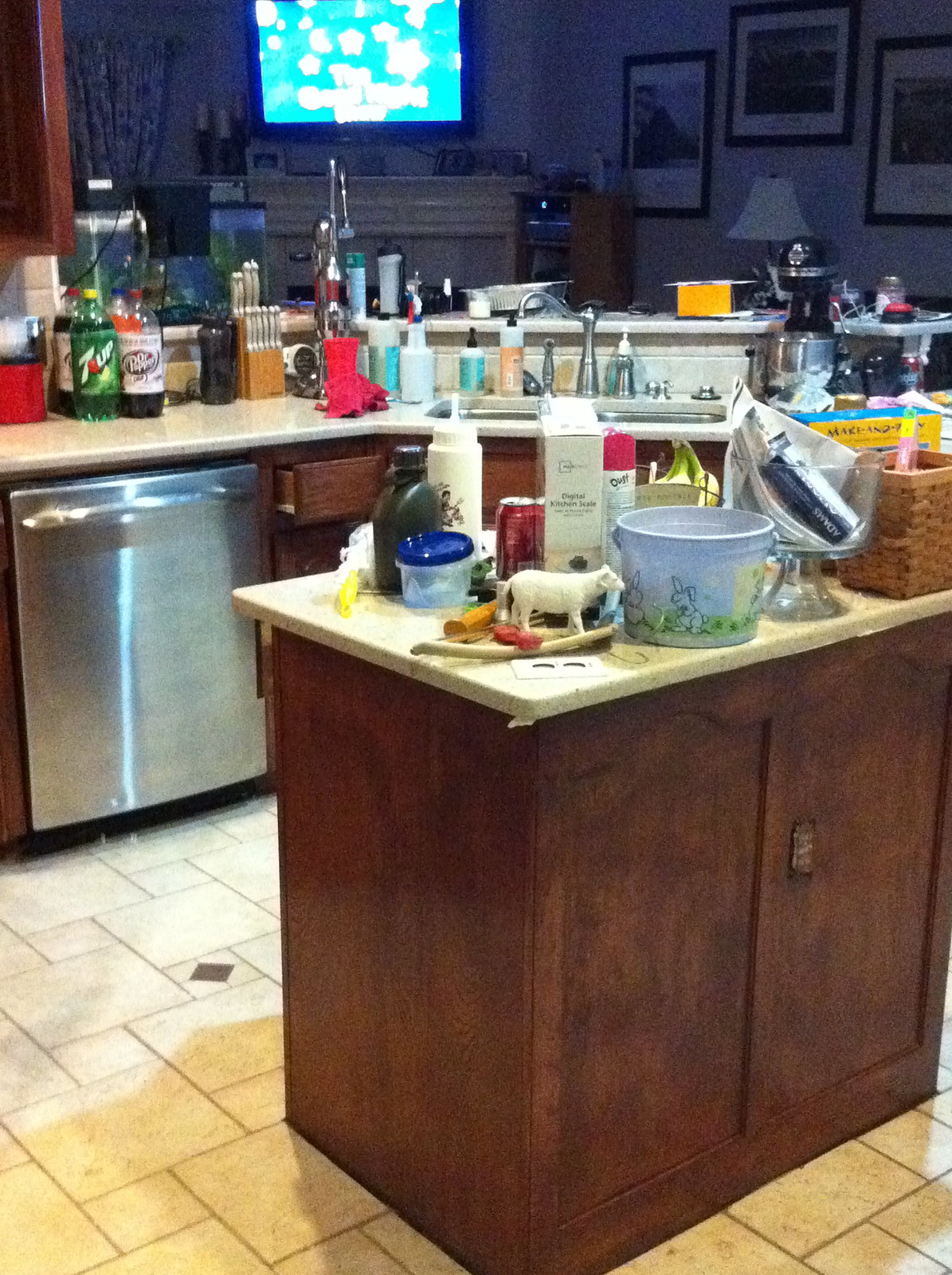This photograph shows an open-concept kitchen seamlessly integrated with a living room area. The kitchen features a wraparound benchtop made of white stone, which overlooks the living room, providing a cohesive and fluid living space. The benchtop is lined with various food items, cooking utensils, cleaning products, and household essentials, suggesting a lively and functional cooking area.

Below the benchtop, there are elegant wooden cabinets that add a touch of warmth and contrast to the kitchen's design. A double kitchen sink is strategically positioned, allowing one to easily engage in meal preparation while simultaneously enjoying the living room's amenities. 

The living room area prominently features a white fireplace with a large flat-screen television mounted above it. The TV screen displays light blue and white imagery, adding a modern touch to the cozy setting. The continuity between the kitchen and living room is emphasized by the absence of any physical barriers, making it possible to watch television while working at the kitchen sink.

The floor ties the space together with its patterned cream-colored tiles, lending a subtle yet sophisticated aesthetic to the overall ambiance.